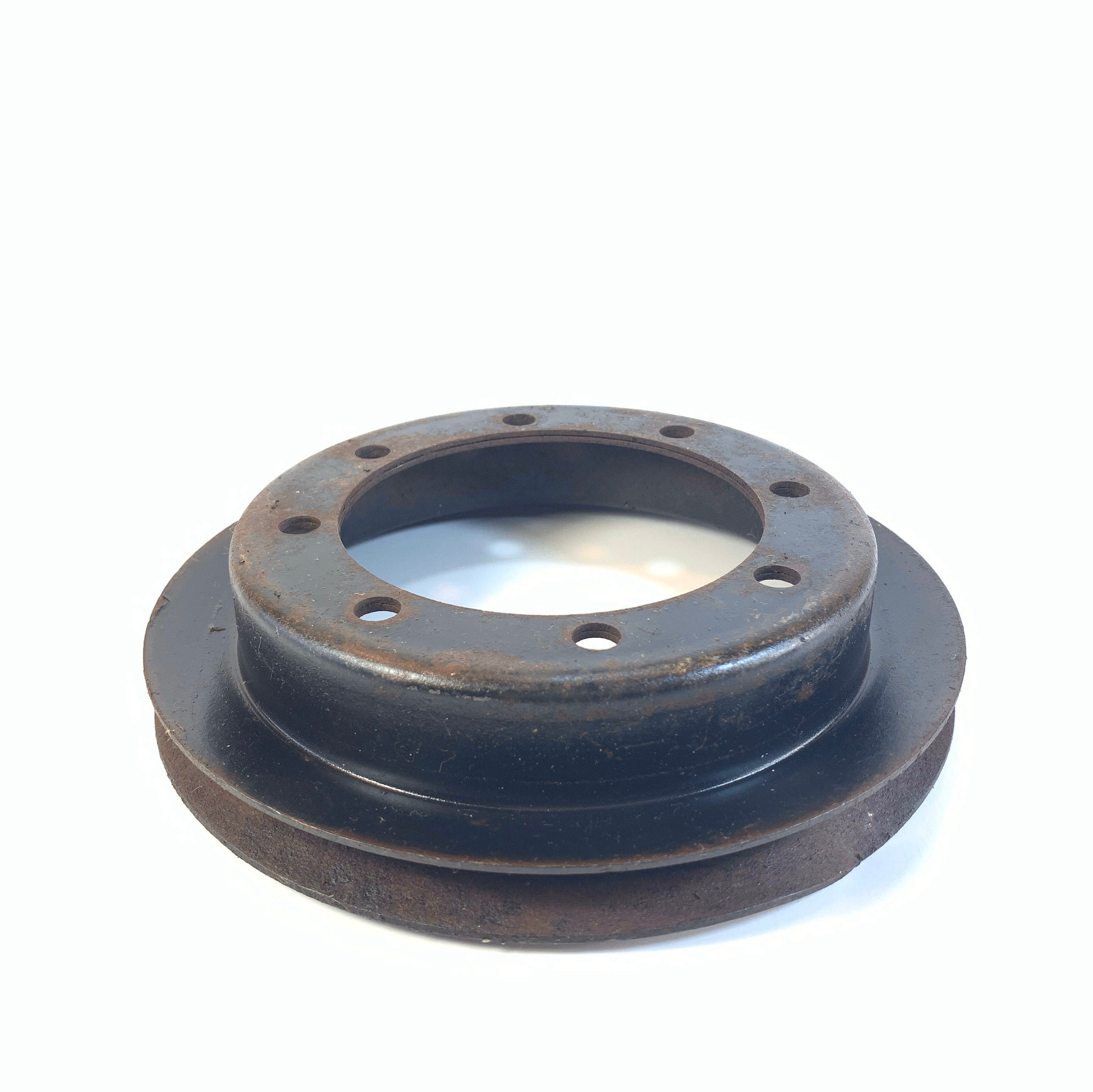The image depicts a dark brown, round metal object that resembles a phalange or hubcap. It features a narrow upper section with a central hole surrounded by eight smaller, evenly spaced holes, through which light reflects onto the white surface below. The object appears to be made of rusted steel, contributing to its brownish tint, and casts a noticeable shadow on the pure white background. The lower part of the object is wider and circular, with indentations suggesting it could be used to wrap or contain something, like a hose. The overall design and structure indicate that it is a piece of hardware, possibly belonging to another tool or object.